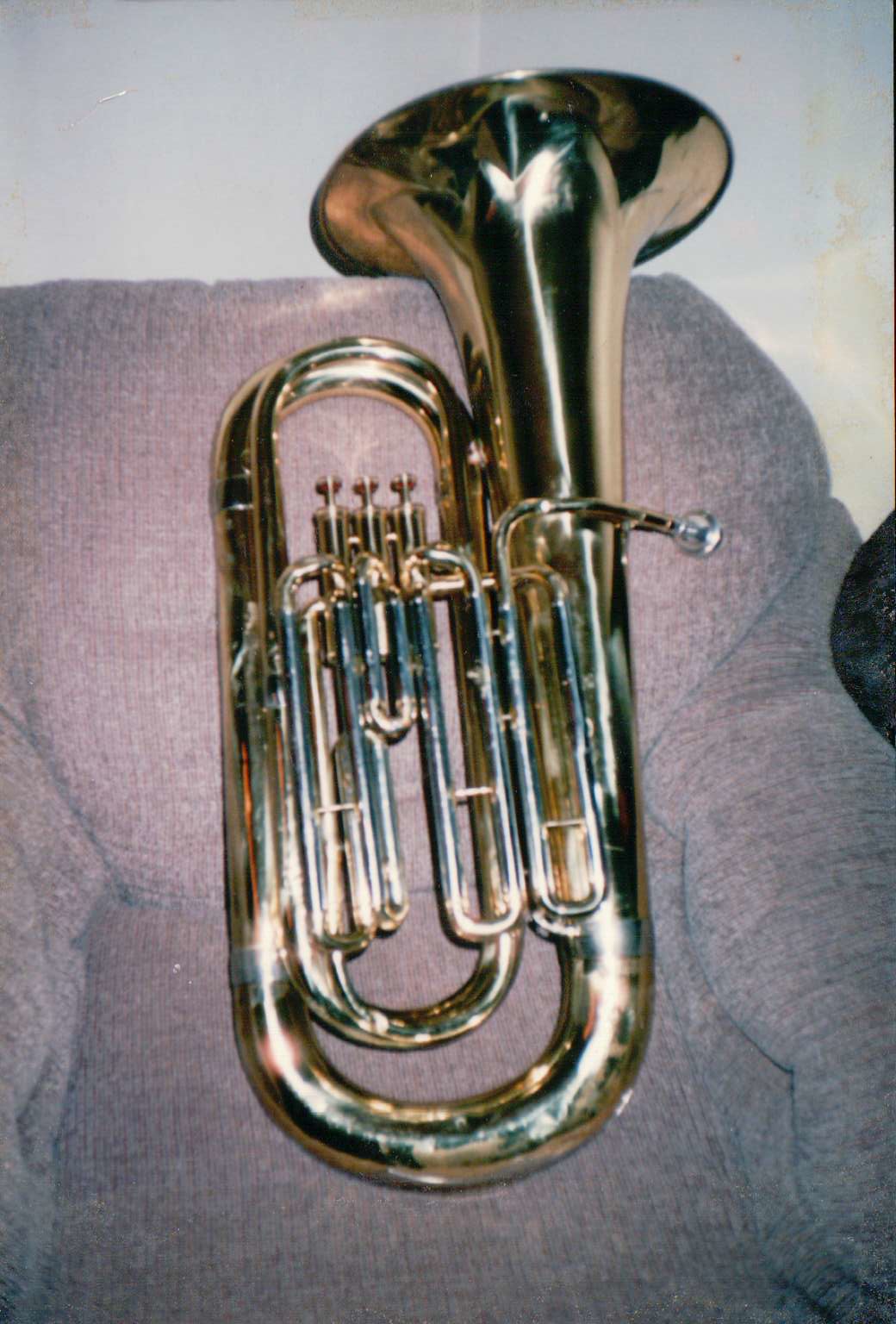The photograph prominently features a large, shiny brass instrument known as a tuba, characterized by its intricate network of coiled tubes, a mouthpiece, and three prominent valves with plungers. The tubing forms a round W shape before expanding into a wide, flared bell at the end. This tuba rests upon an old couch made of tan fabric, illuminated by a flash that causes visible reflections on its glossy golden surface. The couch, appearing somewhat aged, includes a purple cloth draped over it. There are also noticeable dust, scratches, and mold spots on the image, indicative of an old film photograph. The background features a dirty-looking white wall and another partially visible black object, adding context to the setting.